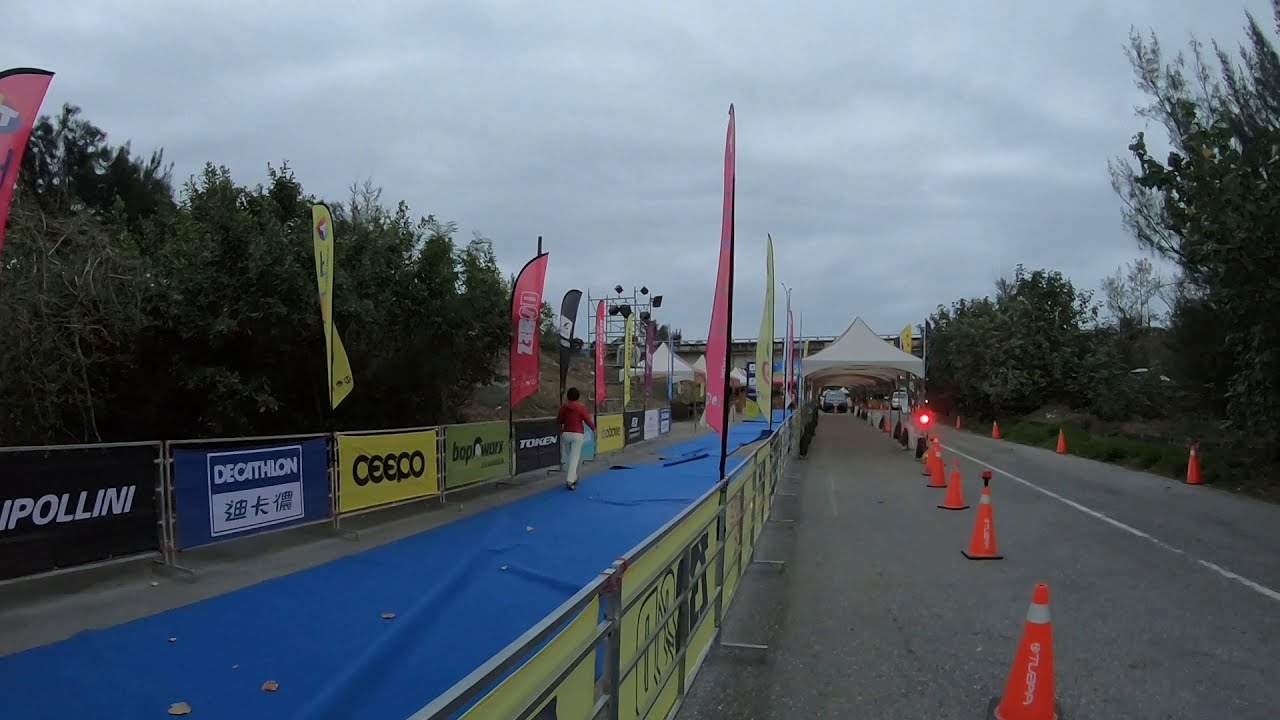The image depicts a two-lane street marked with a white line down the middle, heavily adorned with numerous orange traffic cones lining the left side. A blue tarp stretches along the ground next to barriers that flank both sides of the street, sporting various advertisements, some in Chinese, and flags atop the railings. The scene is set under a gray, cloudy sky, hinting at an overcast day. Trees border both sides of the street, enhancing the outdoor setting with lush greenery. In the distance, white tents are visible, suggesting preparations for a significant event, possibly a race like a triathlon. Near the center of the image, a person in white pants and a red shirt can be seen walking on the blue tarp, contributing to the sense of activity. The backdrop of the image features a bridge and a red light, adding depth to the bustling street scene.